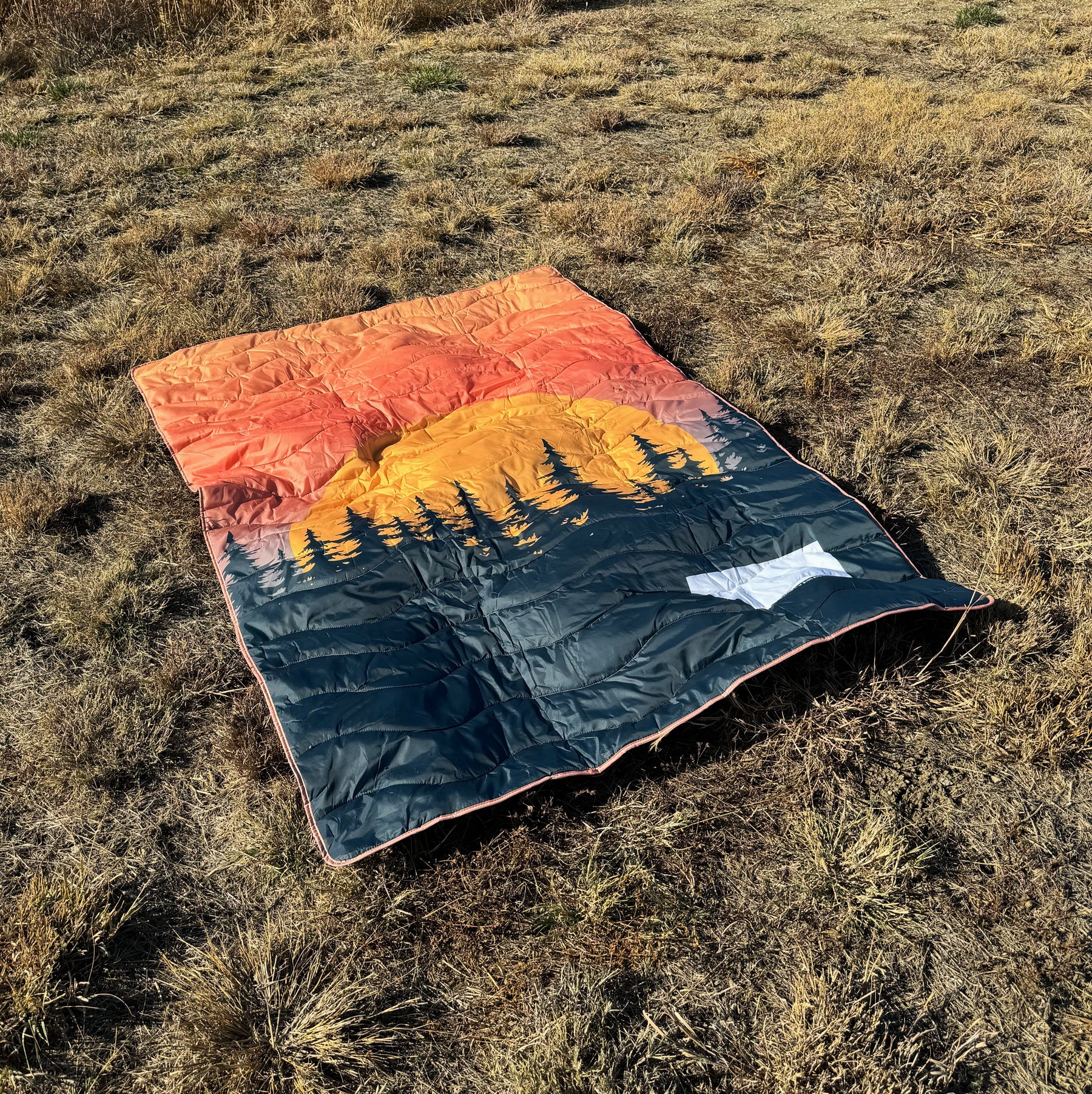In the image, a quilted rectangular blanket lies spread out on the ground, which is covered with patches of dry, yellowish-brown grass, suggesting a high desert field or an area with sparse, struggling plant life. The blanket itself is intricately designed and highly colorful. The bottom section of the blanket is black, transitioning into a middle section adorned with black silhouettes of pine trees. Above the trees, a large yellow half-circle represents the sun, partially hidden behind the treetops. The sky above the sun is richly colored, starting with a light purple hue that blends into reddish-orange, and finally fading into a lighter orange at the top. A blue patch is noticeable in the lower right-hand corner of the blanket. The vibrant and detailed design stands out against the parched backdrop, adding a touch of color to the otherwise dry and barren landscape.